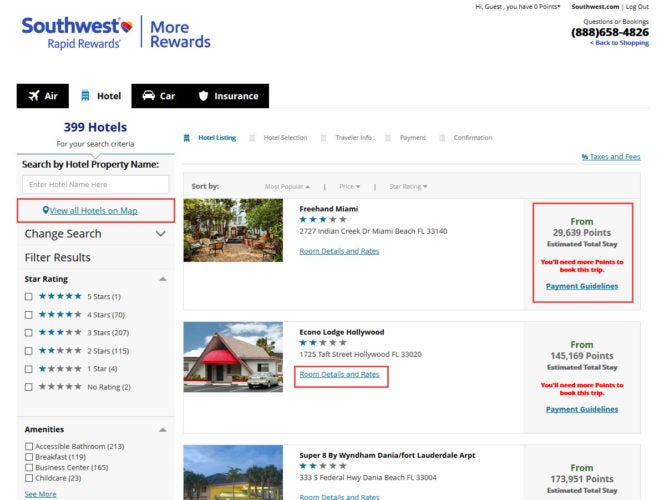A detailed screenshot from the Southwest website, displayed on a desktop. The header shows "Southwest Rapid Rewards" with the "More Rewards" section in the top left corner. On the top right, it states "Hi Guest, you have zero points," alongside options for "Questions or bookings," a contact phone number (888-658-4826), and links for "Southwest.com" and "Logout." A "Back to shopping" link is visible below these options. 

Directly underneath, a navigation menu offers choices for "Air," "Hotel," "Car," and "Insurance" bookings, with the "Hotel" tab currently selected. The screen reports "399 hotels for your search criteria" and provides a search bar to "Search by hotel property name." A red rectangle prominently surrounds a "View all hotels on map" button. Next, a "Change Search" dropdown menu and a "filter results" option are available, which include filters by star ratings and amenities.

On the main section of the page, the search results are displayed. The top result is "Freehand Miami," a three-star hotel situated in Miami Beach. Below that, there are listings for "EconoLodge Hollywood," a two-star hotel in Hollywood, Florida, and "Super 8 by Wyndham," a two-star hotel in Dania Beach, Florida.